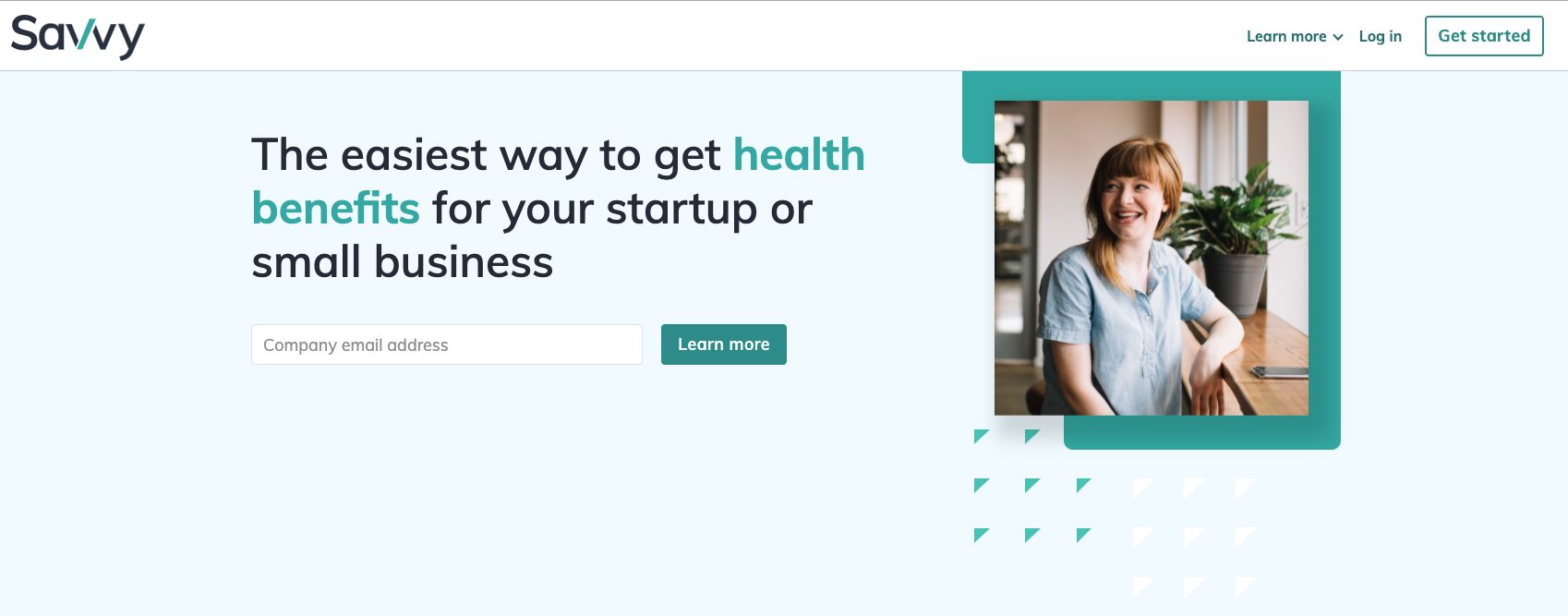The top section of the webpage features the black logo "Savvy," with the right stroke of the first "V" accentuated in blue. To its right, there are navigational options: "Learn More" accompanied by a down arrow, "Log In," and a prominent "Get Started" button. The background transitions into a light seafoam color that fills the remainder of the screen.

Centered in bold black text is the phrase: "The easiest way to get," followed by "health benefits" in blue, and then continuing in black, "for your startup or small business." Below this headline is a small white input box labeled "Company Email Address" and a "Learn More" button in a darker blue box.

On the right side of the screen is a photograph of a smiling woman with light red hair and heavy bangs. She is laughing and looking over her shoulder while resting her hand on a counter. Behind her, there is a plant, and ambient light illuminates the scene from her right. She wears a gray blouse, and on the counter in front of her lies either a tablet or a large cell phone. The image is framed by a darker teal border and features a decorative triangular pattern at the bottom.